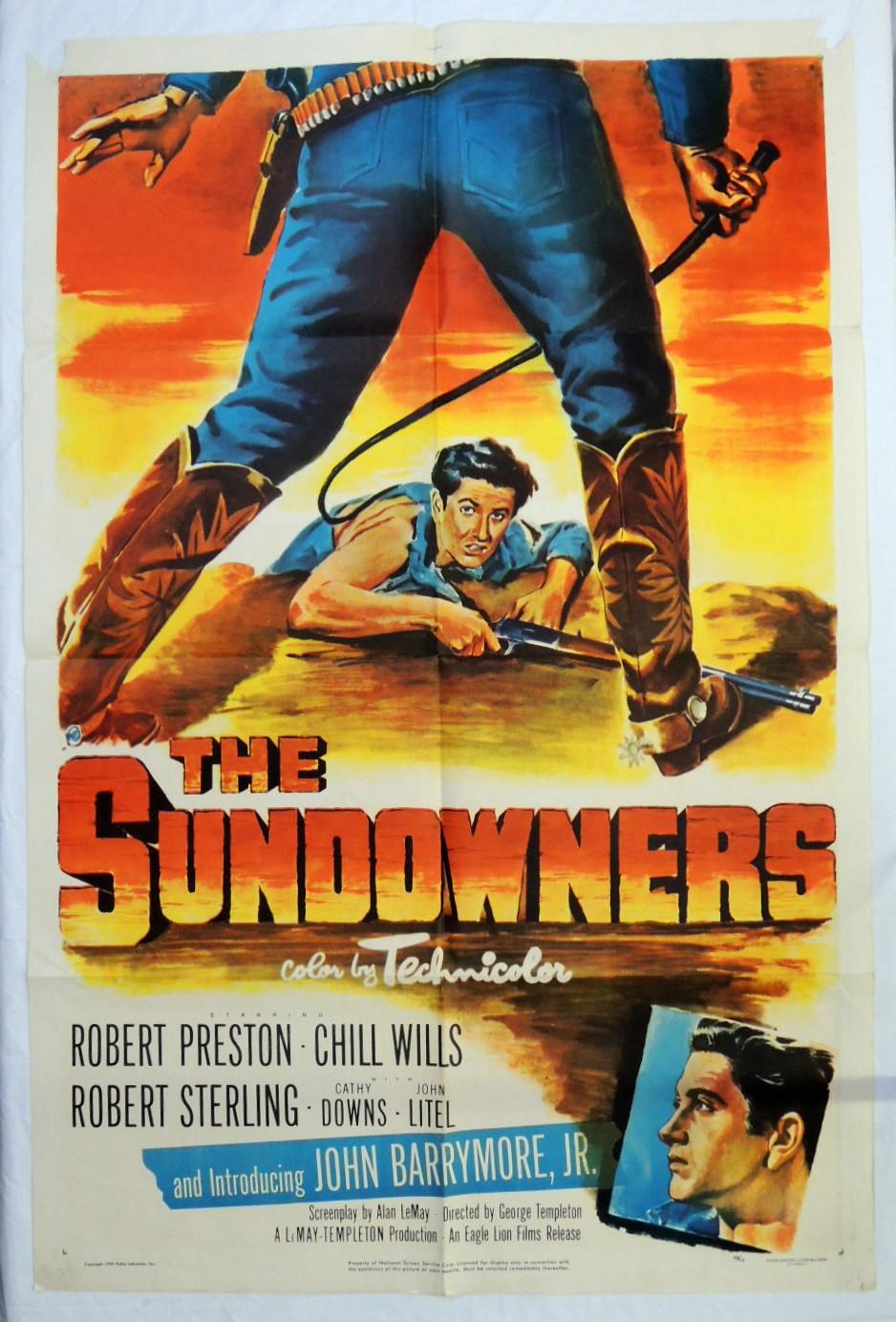This is a detailed and comprehensive caption crafted from the combined input:

The poster is for an old-time movie called "The Sundowners," featuring a distinct yellowed coloring that suggests it’s from the 1940s or 50s. The top of the poster is a reddish hue transitioning into a sunset-like yellow tone, casting an evocative backdrop. Central to the illustration is a dramatic scene: A man with dark, short, combed-back hair clings desperately to the edge of a cliff with his left hand, his blue, torn shirt fluttering. In his right hand, he grips a rifle. His precarious situation is made more intense by another cowboy standing above him, whose face isn't visible, only his back. This man is wearing brown cowboy boots and dark blue jeans, with a bullet-laden bandolier around his waist and a holster at his side. In his right hand, he brandishes a whip, seemingly striking at the man on the cliff.

Beneath this gripping image, the text reads, "The Sundowners," in striking red and yellow, followed by "Color by Technicolor." Further down, in bold, it lists the names of the stars: Robert Preston, Chill Wills, Robert Sterling, Kathy Downs, John Little, and notably introduces John Barrymore Jr., whose illustrated profile is also featured. The text concludes with credits for the screenplay by Alan Millay and direction by George Templeton, representing a LeMay Templeton production released by Eagle Lions.